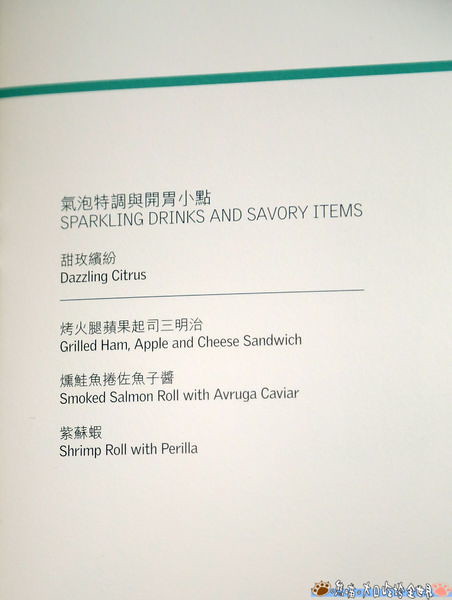The image showcases a text-based menu set against a plain white background. At the very top, a thin green line stretches horizontally from left to right. Below this line, the bilingual text begins, with Chinese (or possibly Japanese) characters followed by their English translations. The English text includes headings and descriptions such as "SPARKLING DRINKS AND SAVORY ITEMS," "Dazzling Citrus," "Grilled Ham, Apple, and Cheese Sandwich," "Smoked Salmon Roll with Avruga Caviar," and "Shrimp Roll with Perilla." The font color appears to be a dark green throughout the menu. Additionally, in the bottom right corner, there's a small cartoon logo featuring a paw print and adjacent Chinese text in white. The paw print is displayed in brown and pink colors.